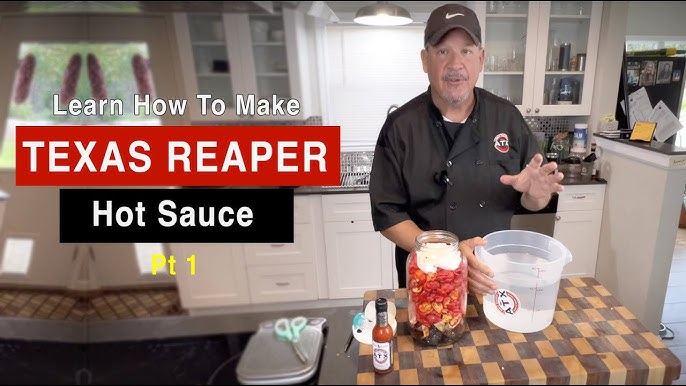The image features an older Caucasian man with a mustache, dark eyes, and a black or gray Nike baseball cap standing in a home-style kitchen. He is wearing a black short-sleeved chef's shirt with a letter 'T' logo on the left side, and a microphone is clipped to the shirt. The kitchen has white wooden cabinets with glass windows above the countertop, a sink, and a window with a light above it.

The man is positioned behind a butcher block counter characterized by a dark and light brown checkerboard pattern. On the counter, there is a large clear plastic pail of water, a big clear glass jar filled with chopped red, yellow, and black peppers, presumably dried, and a bottle of hot sauce. The man appears to be talking to a camera, possibly recording a tutorial.

To the left of the man, text in white reads "Learn how to make," followed by a red banner with "Texas Reaper" in white capital letters, and a black banner below it with "hot sauce" written in white. Below this, "Part 1" is displayed in yellow text. This image is presumably a thumbnail for a video tutorial on making Texas Reaper hot sauce.